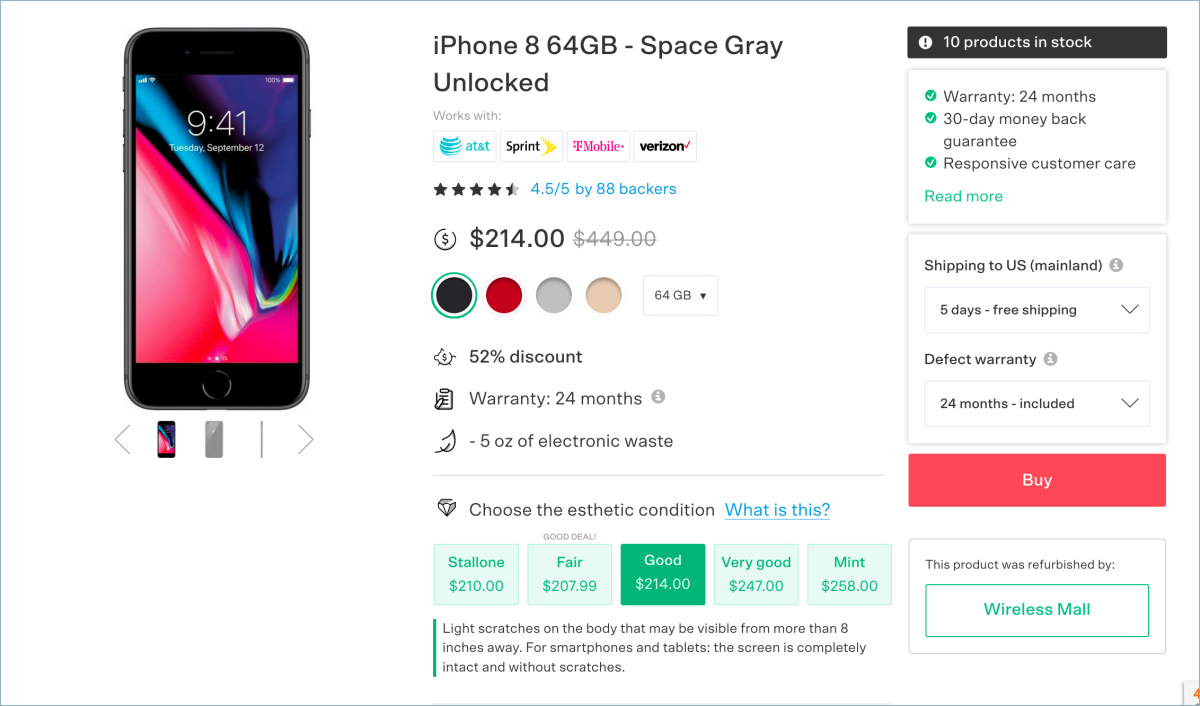This screen grab showcases an iPhone 8 available for purchase. The specifications of the phone include 64GB of storage, a space gray color, and it's unlocked, making it compatible with carriers such as AT&T, Sprint, T-Mobile, and Verizon. It boasts a user rating of 4.5 out of 5 stars based on reviews from 88 backers. The current price is $214, marked down from the original price of $499, reflecting a 52% discount. 

Beneath the price, there are options to select from four different colors and a dropdown menu for choosing the preferred storage capacity. The phone is noted to have been manufactured using 5 ounces of electronic waste. Customers can choose the aesthetic condition of the device, with the following price options: Stallone ($210), Fair ($207.99), Good ($214), Very Good ($247), and Mint Condition ($258). 

On the left-hand side of the screen grab, there is an image of the iPhone, while additional details are provided on the right-hand side. These details confirm that there are 10 units currently in stock. The purchase includes a 24-month warranty, a 30-day money-back guarantee, and responsive customer service. Shipping options within the U.S. are also shown, including 5-day free shipping.